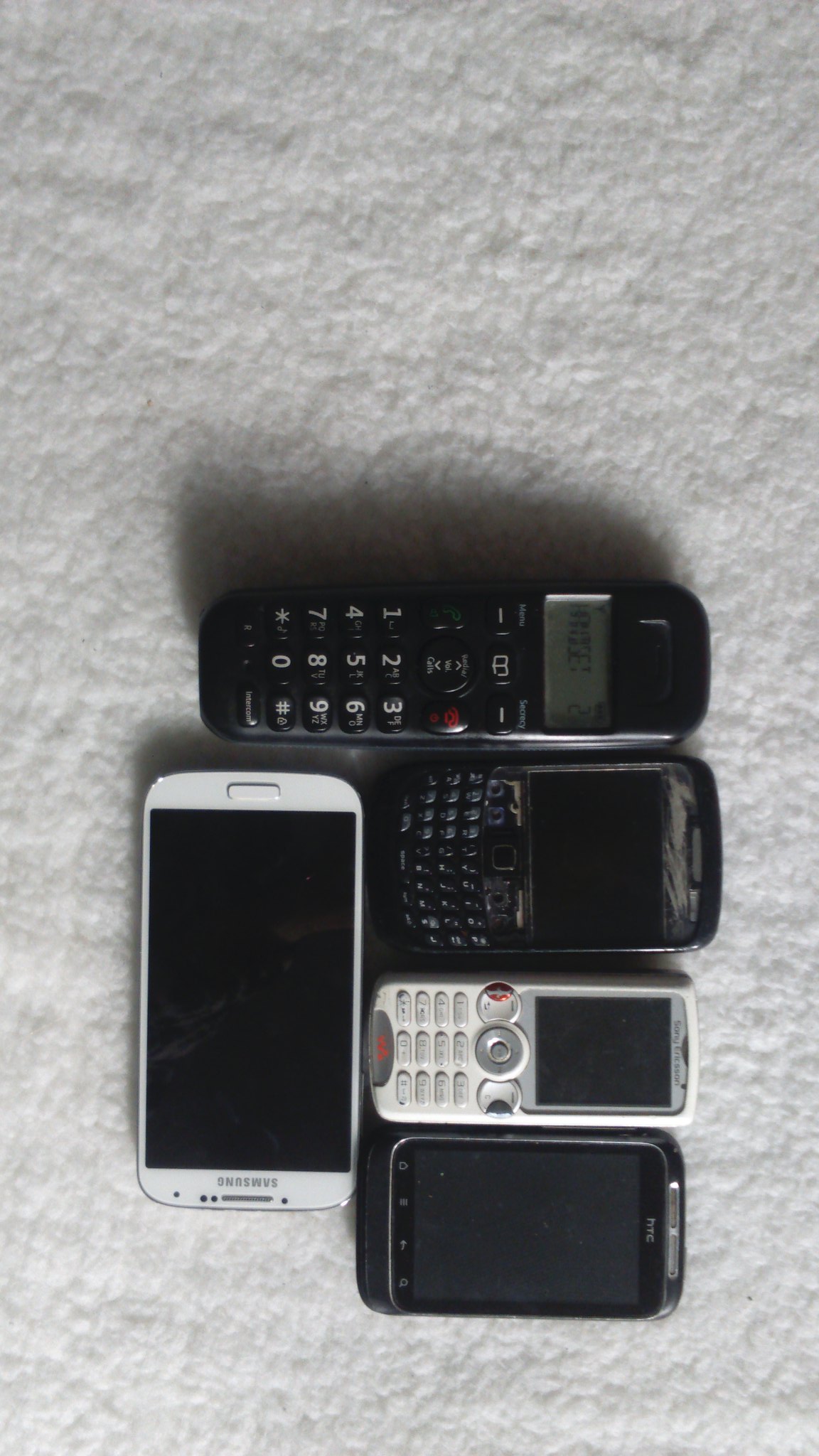This image, taken from an overhead perspective in portrait mode, features five cell phones placed on a bright, pure white, fluffy surface, possibly made of fleece, carpet, or a bedspread. The phones are arranged in a slightly irregular pattern: a single white Samsung smartphone with a black screen, gray "Samsung" text at the top, and a vertically oriented position on the left side. To the right of it, in a horizontal alignment from top to bottom, are four other phones. The topmost is a black device resembling either a traditional feature phone or a landline handset with a small screen and black buttons. Below it sits a scratched BlackBerry with a large square screen and black and gray buttons. Next in line is an older, small white phone with a small screen and white buttons, brand unspecified. The bottommost phone is a black HTC model marked by gray text at the top, featuring a large screen and designed to slide up to reveal physical buttons. The minimalistic background ensures all focus remains on the differing ages and designs of the phones.